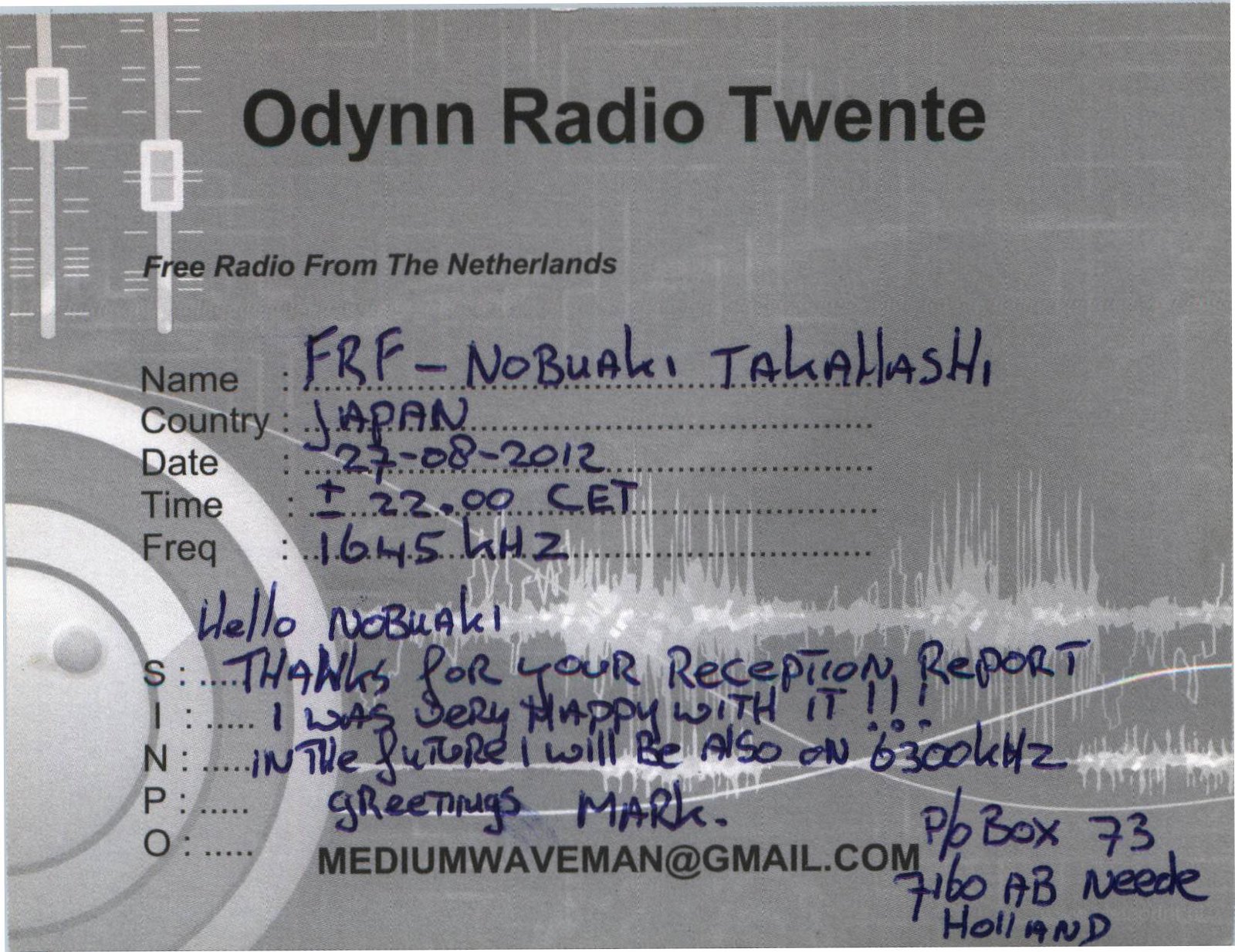The image is a wide rectangular form filled out by hand, with a grey background that features a faint white crisscross pattern. Adorning the top left corner is an illustration of radio dials, and the bottom left corner shows the edge of a circular dial. On the right side towards the bottom, there is an image depicting static in white and grey. The top of the form bears the heading "Oden Radio Twente" in bold black text, followed by "Free Radio from the Netherlands" in italic font. Below this, the form contains a series of dotted lines with the labels: "Name," "Country," "Date," "Time," and "FREQ," and beneath these, more dotted lines are labeled "SINPO." The form is filled in with the following details: Name: FRF Nobuaki Takahashi, Country: Japan, Date: 27-08-2012, Time: 22:00 CET, and Frequency: 1645 kHz. At the bottom, there is a handwritten message that reads, "Hello Nobuaki, thanks for your reception report. I was very happy with it. In the future, I will also be on 6300 kHz. Greetings, Mark." Additionally, the form provides a P.O. Box address in Holland and an email address, mediumwaveman at Gmail.